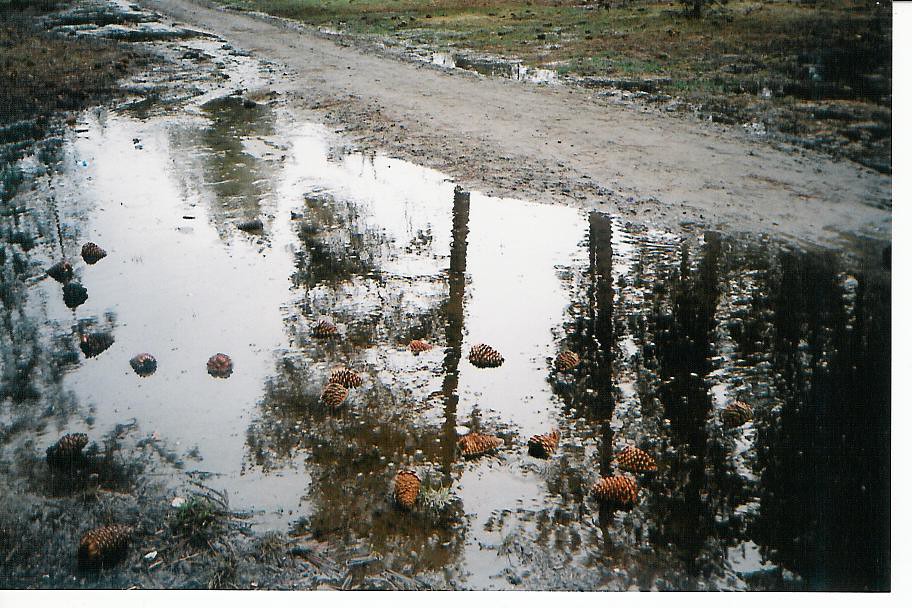This photograph captures the aftermath of a heavy rainstorm along a dirt path adjacent to a flooded roadside area. The scene is dominated by a large, reflective puddle bordered by mud and patches of wet grass. In the puddle, several light brown pine cones float on the water's surface, their various shades of brown contrasting against the murky water. The water is not very clear, but it mirrors the tall pine trees and the overcast, white sky above, adding depth to the composition. A few pine cones remain perched on the mud near the bottom left of the frame, unaffected by the flooding. Raindrops can be seen creating ripples in the puddle, emphasizing the ongoing drizzle.